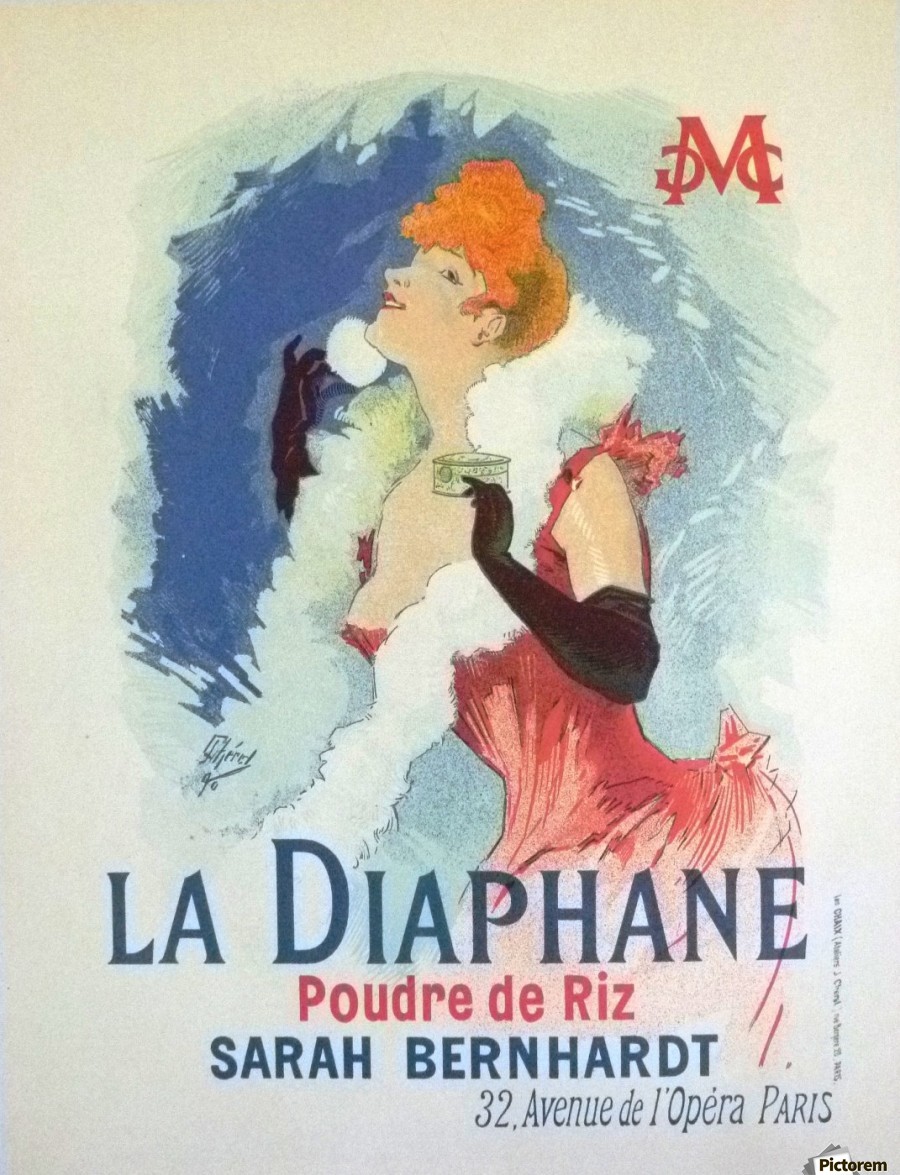The poster is an advertisement for an opera or play titled "La Diaphane," likely targeting a French-speaking audience, as the text and details are in French. The featured actress in the play is Sarah Bernhardt. The action seems to take place at 32 Avenue de l'Opéra, Paris, possibly under the direction of Paudre de Ries. The bottom right corner of the poster contains the logo "Pictorum," which might be the service that produced the illustration.

The poster illustrates a vibrant, colorful, drawn image of a dramatic scene from the 1920s. The focal point is a woman with a distinctive short mass of orange-red hair tufted over her forehead, meticulously depicted as she applies makeup. Dressed in a red, low-cut showgirl costume that is tied behind her waist, she also dons very long black gloves extending past her elbows. A long, flowing, white fur scarf drapes around her, adding an element of elegance to the composition. She is holding what appears to be a makeup tin in one of her gloved hands, and she uses a white cotton or fur puff to powder her face. Her gaze is directed towards the ceiling with her eyes subtly cocked towards the viewer, adding a captivating and engaging element to her pose. The background features splashes of blue and light blue against a white vignetted frame, creating a contrast that highlights her figure. 

Text elements include "La Diaphane" prominently at the bottom in blue, with additional red text featuring "Poudre de Ries, Sarah Bernhardt, 32 Avenue de l'Opéra Paris." In the top right, a stylistic touch shows letters M, C, and a backwards G interwoven, adding to the visual interest of the poster.